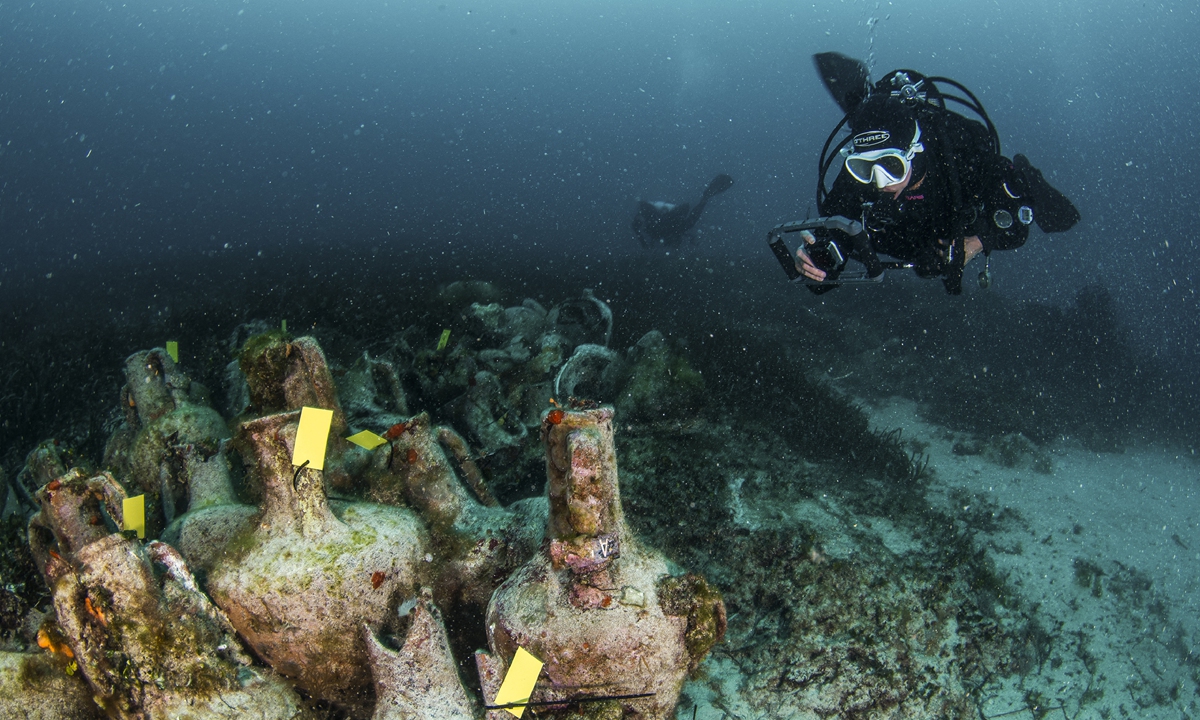In this captivating underwater scene, a diver clad in robust black diving gear and a silver-colored mask explores the depths of a deep, dark blue ocean. Tiny bubbles rise around him as he navigates with a black camera in one hand. A dark-colored fish swims nearby, adding to the aquatic ambiance. The ocean floor is visible, adorned with lush green plants and various rocks. Among these natural elements lie numerous ancient pottery pieces, each displaying a reddish hue interspersed with white, ashy, and green patches. Notably, every piece of pottery is marked with a yellow tag, indicating their significance.